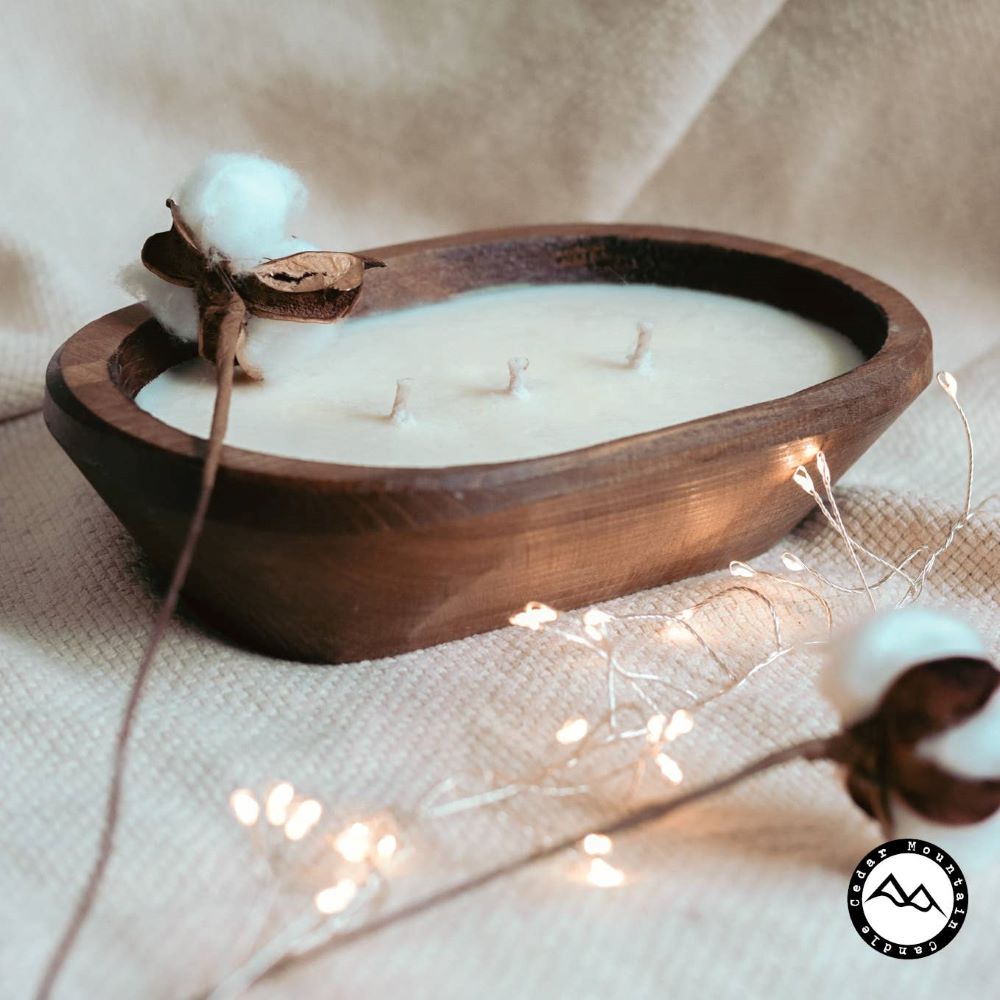This close-up image showcases a handcrafted, milky white three-wick candle set inside an oval, dark wooden bowl that resembles a mini-bathtub. The candle, slightly smaller than a hand, sits gracefully on an off-white, burlap-like fabric that continues behind it, serving as a backdrop. Adorning this scene are delicate fairy lights spread out in front of the candle, enhancing its charm. Complementing the rustic elegance, a cotton stem lies on the edge of the bowl, while another cotton stem is laid out in front of it. The bottom right corner subtly features the Cedar Mountain Candles logo, blending seamlessly with the serene and cozy ambiance of the white burlap fabric backdrop.